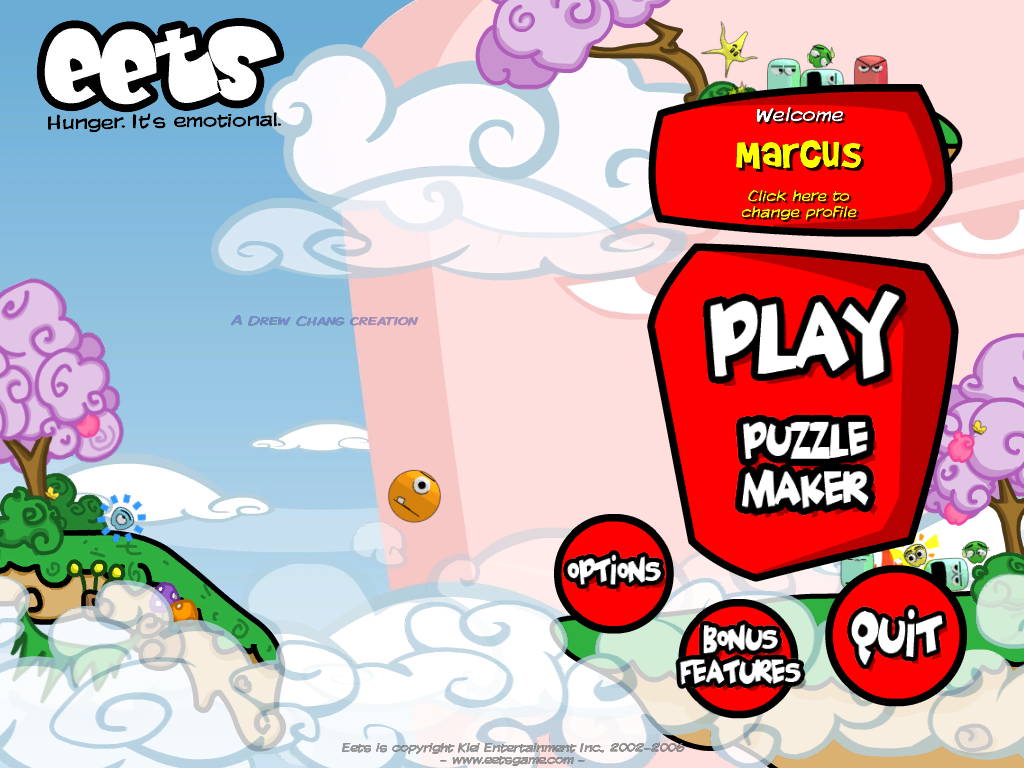A screenshot from a mobile game is displayed, featuring a visually appealing background that transitions from baby blue on the left to an image of a Caucasian figure on the right. This figure is characterized by two white eyes with dark black irises and white hair outlined in black. On the upper left side of the image, white text outlined in black reads "EETS," while below it, in black text, it says "Hunger: it's emotional."

In the lower left section, there's a visually interesting purple tree with a black trunk, surrounded by green grass and a cluster of clouds at the bottom. On the right side, another similar tree is visible. Further to the right, a rectangular box warmly welcomes the user with the text "Welcome Marcus" in white, where "Marcus" is highlighted in yellow, followed by the instruction in yellow, "click here to change profile."

Below this, another box presents the options "Play" and "Puzzle Maker" in white text. Beneath these, three black circles with white text offer additional options: "Options," "Bonus Features," and "Quit." Despite the detailed visuals, the narrator expresses a dismissive view of the game, suggesting it is likely unpopular and not very engaging.